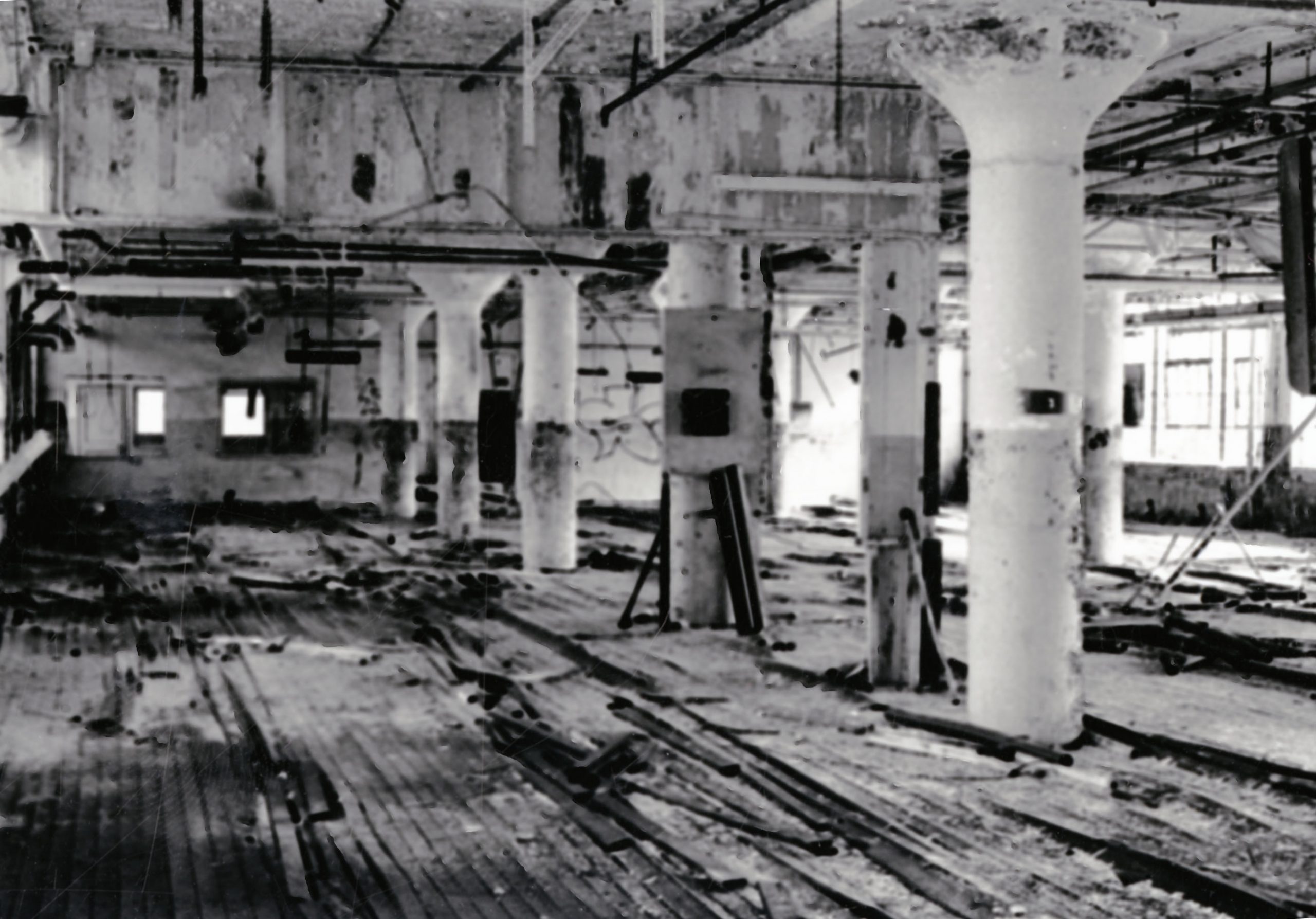This is a black-and-white photograph depicting the interior of an old, decrepit warehouse in significant disrepair. The scene is characterized by shades of gray, black, and off-white, giving it a dingy, abandoned look. The large, open space features a wooden plank floor, with many floorboards buckled, broken, or missing, suggesting extreme neglect and decay. Central to the composition, a row of six large, white concrete pillars extends from the foreground to the background, supporting what appears to be a high, 15-foot metal or cement ceiling. The ceiling shows signs of damage, with paint peeling and the presence of rusted pipes and hanging cables. On the right-hand side, bright daylight pours through numerous large, open windows, accentuating the absence of any artificial lighting. To the left and in the background, smaller open windows or holes reveal further structural damage and exposure to the elements. The walls and overall structure have sustained substantial damage, indicative of either long-term abandonment or possibly a past disaster such as a fire. The scene is littered with debris, enhancing the overall sense of desolation and historical neglect.